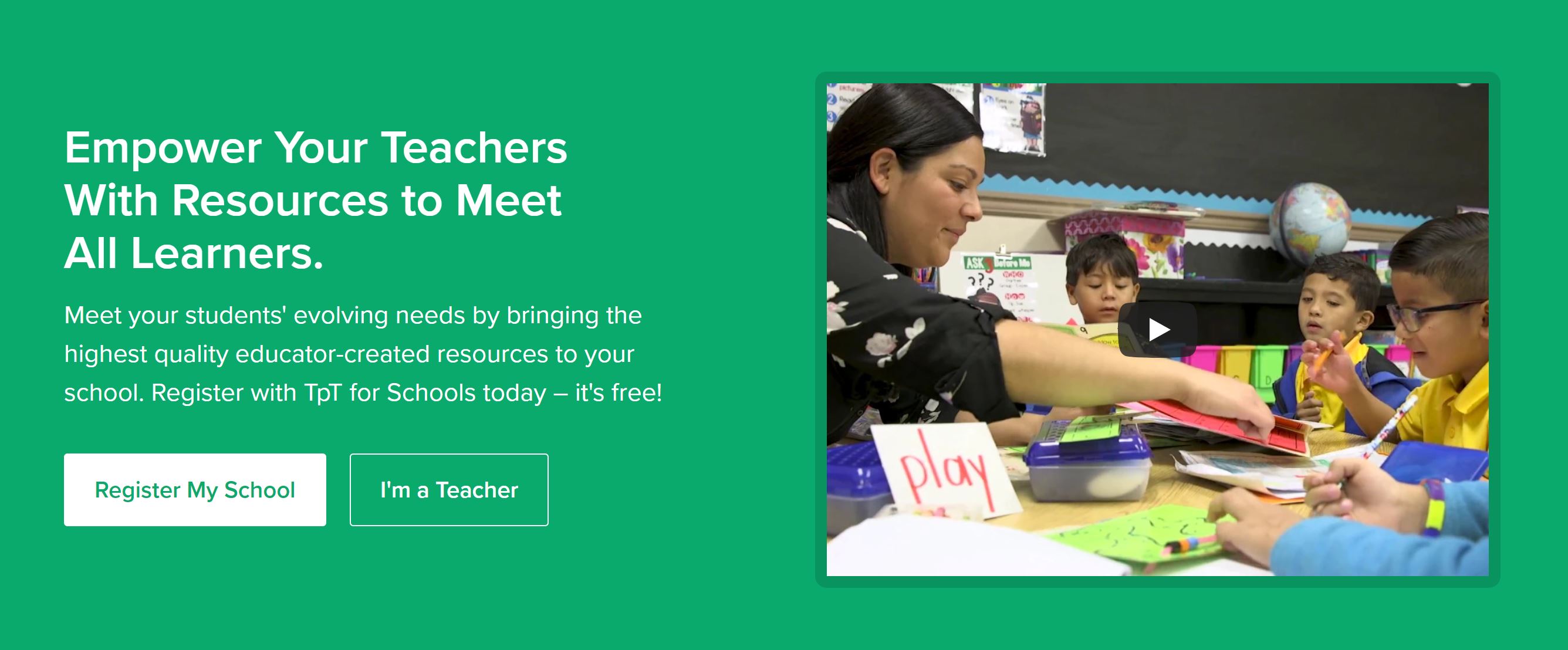The image is a desktop screenshot featuring a promotional banner for TPT (Teachers Pay Teachers) for Schools. The background of the banner is a medium to pale green rectangle. On the left side, in large white print, the banner reads: "Empower your teachers with resources to meet all learners." Below this, in smaller white print, it continues: "Meet your students' evolving needs by bringing the highest quality, educator-created resources to your school. Register with TPT for Schools today. It's free."

At the bottom of the left section, there are two call-to-action buttons. The first is a white rectangle with green text that says "Register My School." The second is a green rectangle with white text that says "I'm a Teacher."

On the right side of the banner, there is a video still featuring a classroom scene. In the foreground of the video, a woman with medium brown skin and black hair, likely a teacher, is pointing something out to her students. The classroom environment includes a large chalkboard/blackboard and a globe in the background. The students visible in the image are boys with medium brown skin and brownish-black hair. On their table, various educational supplies such as pencils, construction paper, and containers are scattered.

This detailed classroom scene supports the messaging of the banner, illustrating how TPT for Schools aims to provide high-quality educational resources to empower teachers and meet diverse student needs.